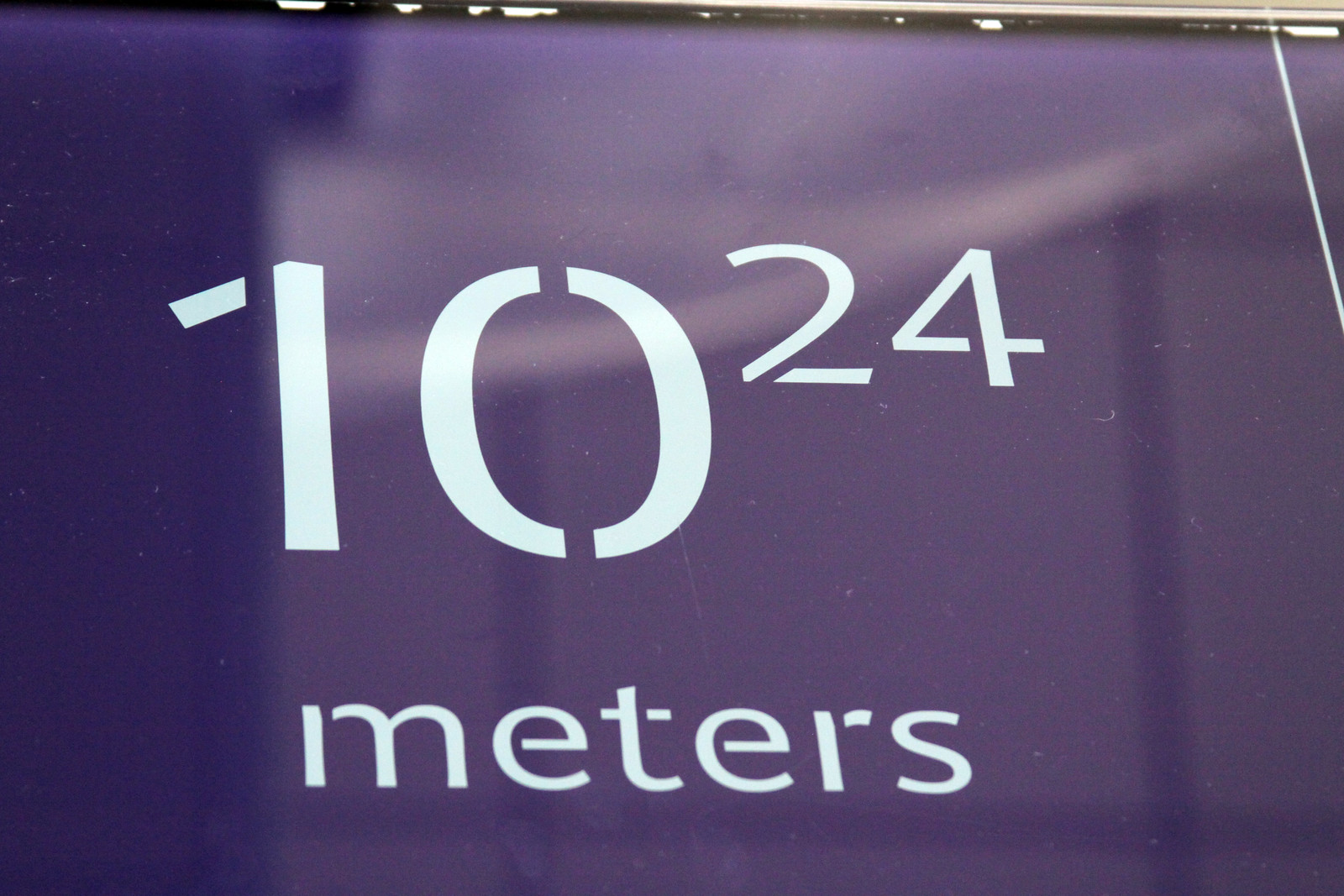The image depicts a shiny plastic or metal sign set against a background that appears purple. The sign prominently features the text "10 to the 24 meters" in white block stencil-like letters. The number "10" is larger, with "24" positioned slightly above and to the right of the zero in a smaller font. There's a subtle reflection on the surface of the sign, suggesting it is glossy, and a vertical white line can be seen in the top right corner. The very top of the sign shows signs of wear, with what looks like chipping or peeling paint. The setting appears to be outdoors, given the natural light reflected on the sign, and there's a possibility that the sign could be part of a street or pool marking, although its exact purpose remains unclear. Additionally, parts of the background hint at a white surface and black table legs.